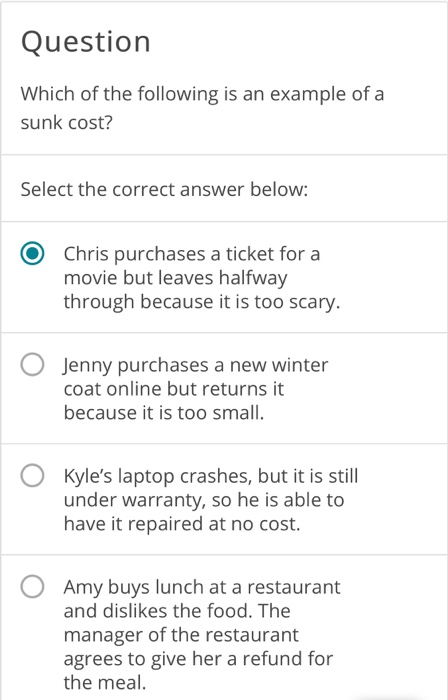The image depicts a question page with a clearly structured layout. At the top left corner, it says "Question," followed by the query: "Which of the following is an example of a sunk cost? Select the correct answer below." The options are neatly organized in a chart format with thin gray lines separating each choice. 

The first option is highlighted with a green target symbol comprising a green dot at the center and a green circular outline around it. It reads: "Chris purchases a ticket for a movie but leaves halfway through because it is too scary."

The second option, delineated by a gray circle, states: "Jenny purchases a new winter coat online but returns it because it is too small."

The third option says: "Kyle’s laptop crashes, but it is still under warranty, so he was able to have it repaired at no cost."

The final option reads: "Amy buys lunch at a restaurant and dislikes the food. The manager of the restaurant agrees to give her a refund for the meal."